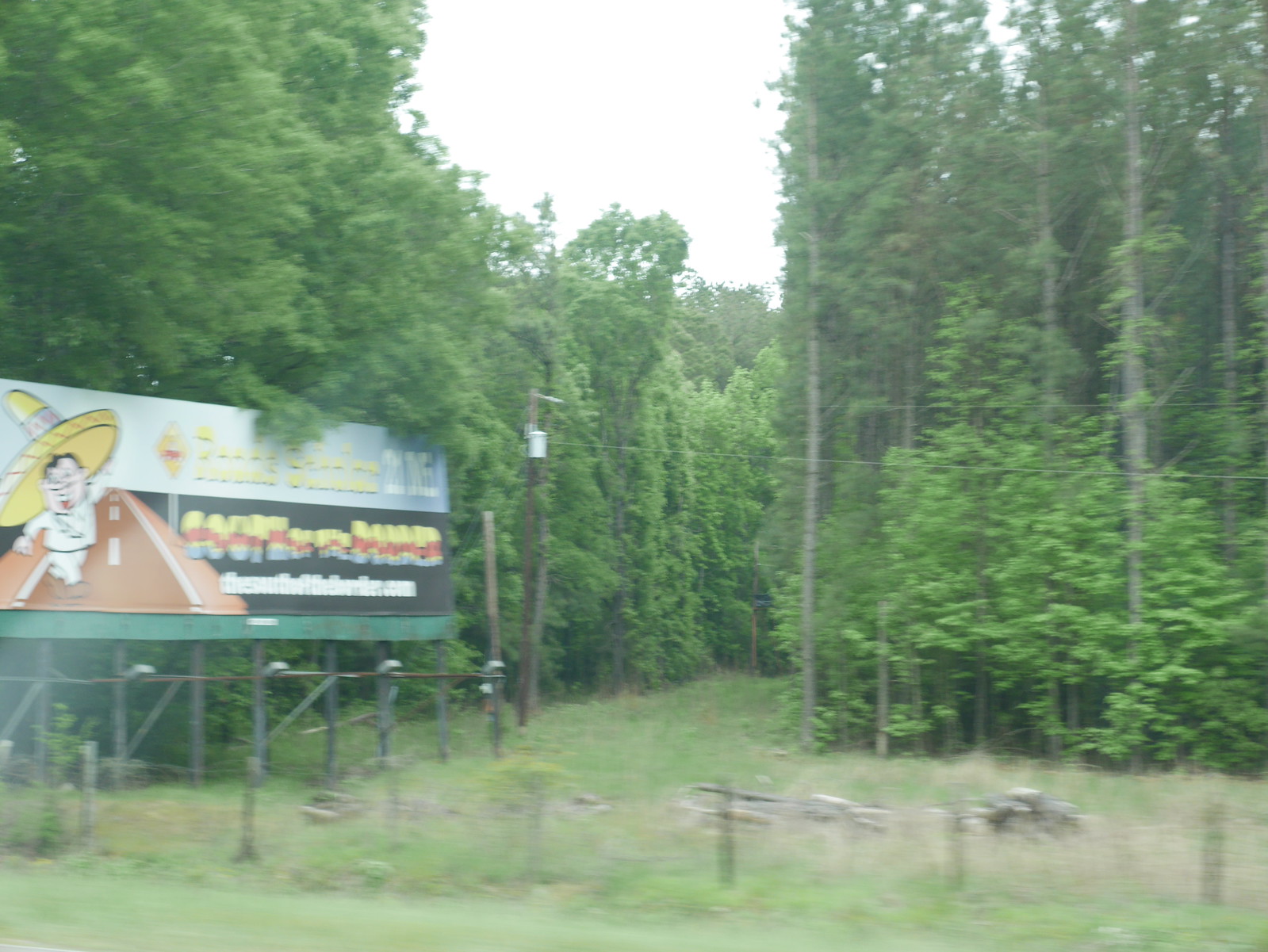The image depicts a dense forest area with numerous tall trees, their lush branches forming a green canopy overhead. Amidst the foliage, a winding pathway can be seen, meandering through the trees and partially obscured by grasses and undergrowth. In the foreground, there are rustic wooden fences, which add to the natural, unspoiled ambiance of the scene.

On the left side of the image, a prominent billboard stands out featuring an illustration of a Mexican individual donning a traditional sombrero. The character is dressed in a pristine white suit and matching white pants, complemented by brown shoes. He is depicted standing confidently on a brown-colored highway. Although the right side of the billboard is difficult to decipher, it appears to be advertising a restaurant, providing directions and the exit to take to reach the establishment. The overall scene exudes a blend of natural tranquility and subtle commercial presence, inviting both exploration and curiosity.